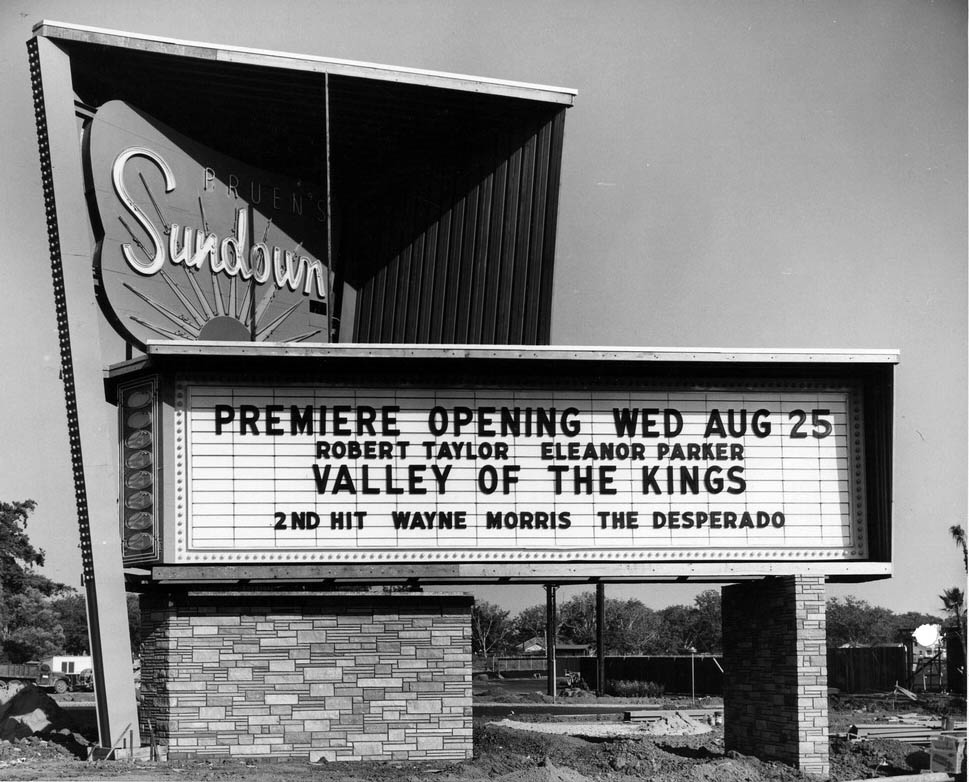The black-and-white photograph depicts a nostalgic and defunct drive-in movie theater named "The Sundown." Dominating the scene is a large, brick-walled marquee, typical of classic drive-ins. The marquee proudly advertises its premiere opening held on Wednesday, August 25th featuring "Valley of the Kings" starring Robert Taylor and Eleanor Parker, and a second feature, "The Desperado" starring Wayne Morris. The marquee is detailed with lights around its edges and crowned by the theater's name "Sundown" alongside a depiction of a half sun with radiating spikes, emblematic of vintage designs. This image, with its abandoned background, evokes a poignant sense of nostalgia, emphasizing the bygone era of once-popular drive-in movie theaters.